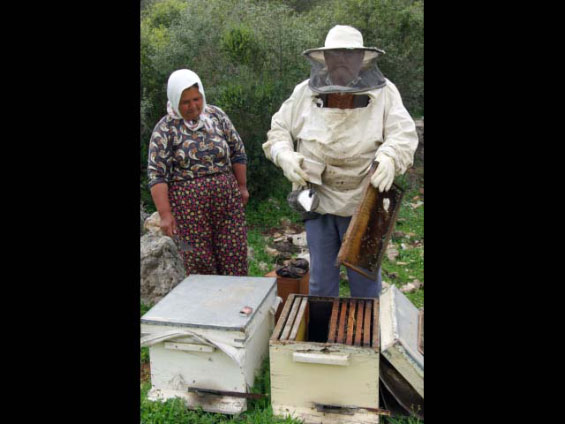The photograph depicts an outdoor scene featuring two people and beekeeping equipment on a grassy field with trees in the background. On the right side stands a man dressed in a full beekeeping suit, complete with a white hat, gray mesh netting over his face, and white gloves. He is wearing jeans and holding a wooden honeycomb frame he has just removed from one of the beehive boxes in front of him. The box on the right is open, revealing multiple honeycomb frames inside, while the box on the left remains sealed but is identical in size and shape, suggesting it also contains honeycombs. To the left, a woman is positioned behind the closed box. She is dressed in colorful trousers with a pattern of black, yellow, and red dots, a patterned gray blouse with rolled-up sleeves, and a white headscarf. The lush greenery of grass and trees forms the backdrop, adding a natural and serene setting to the beekeeping activity. The photo appears to be taken vertically, leaving black margins on both sides due to the aspect ratio.